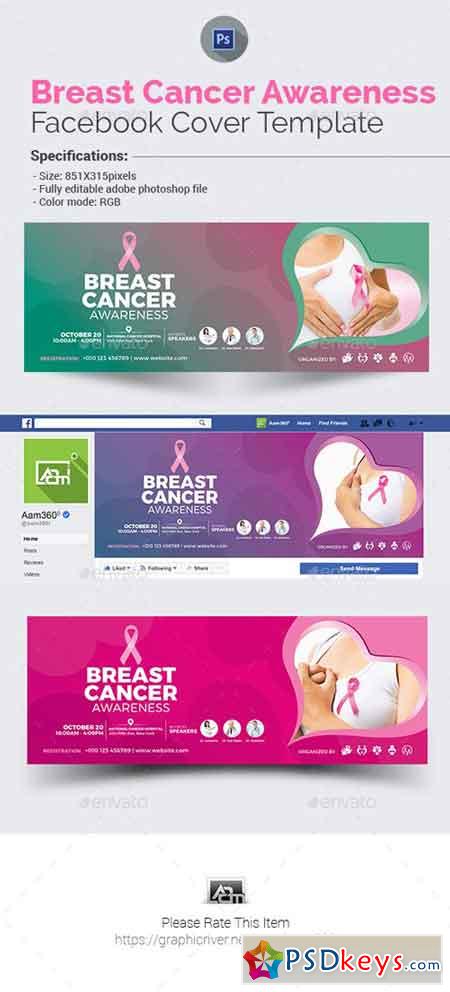This image appears to be a composite screenshot possibly created on a mobile device. It showcases various design elements, seemingly related to Breast Cancer Awareness and a digital template.

At the top of the image, there is a light pink background with a centered, darker blue box. Inside this box, there is a purple square with white text reading "PS". Below this, in pink text, it says "Breast Cancer Awareness", and underneath, in black text, it reads "Facebook Cover Template".

Further details include specifications listed in black text: "Size: 815 by 318 pixels", "Fully editable Adobe Photoshop file", and "Colour mode: RGB". A dividing line extends to the right, separating the specifications from additional elements.

On the right side of the image, there are three sections vertically aligned, each featuring a heart with a woman holding her breast adorned with a pink ribbon, symbolizing Breast Cancer Awareness. Adjacent to these sections, on the left, there is repeated text in white within a purple/pink background that reads "Breast Cancer Awareness".

In the center, slightly towards the left, there is a section with a green element and more text below it, which in black text on a white background reads "Please Rate This Item". Overlaid on the entire bottom part of the image is a gray-colored layer with the website "PDSKeys.com" written in black text.